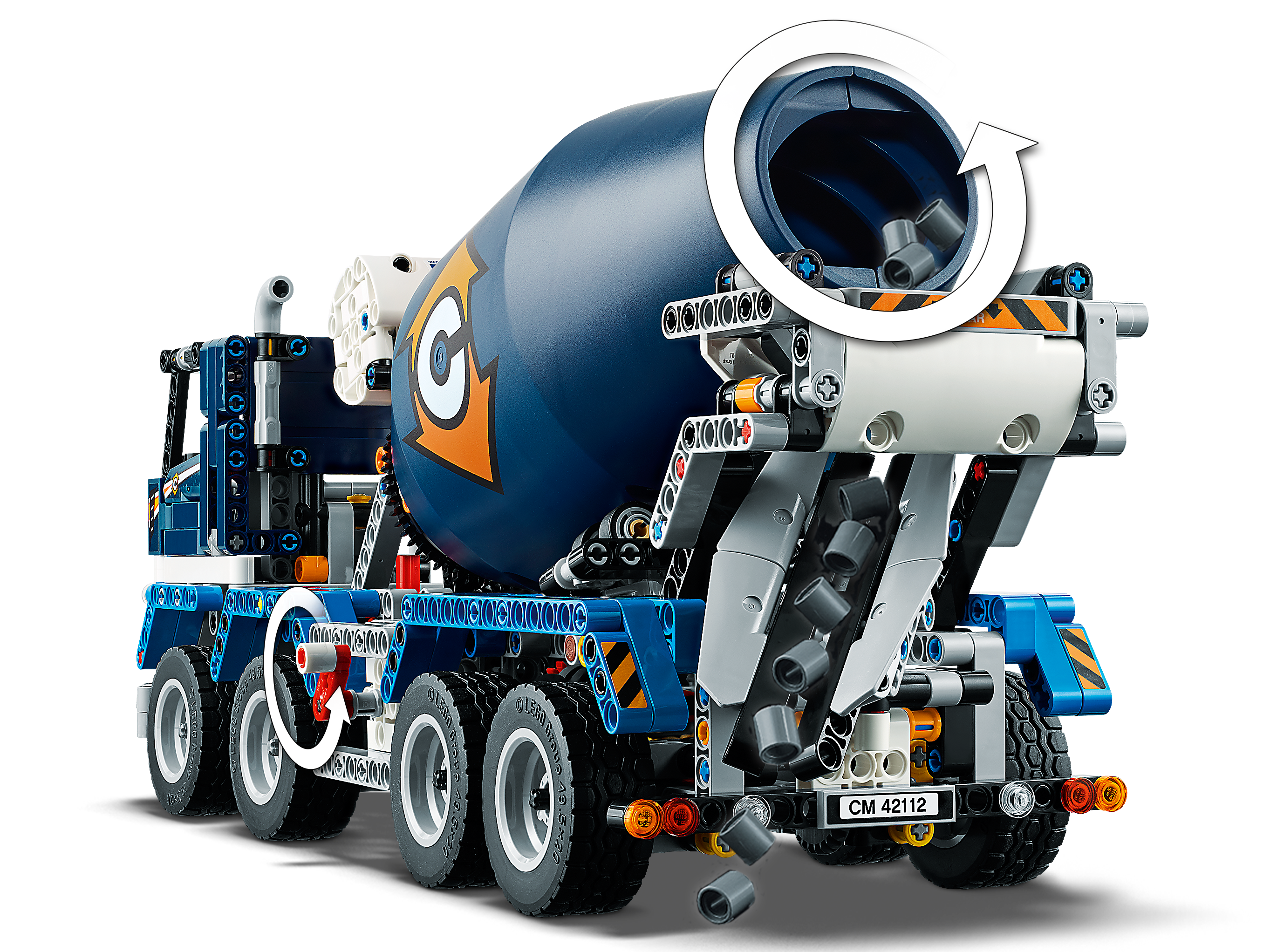This image features a highly detailed 3D rendition of a Lego cement mixing truck. The truck is primarily dark blue with a cylindrical mixing drum at the back, also in dark blue, adorned with a distinct gold arrow pointing up and down. Centrally overlaid on this arrow is a large white 'C'. At the entrance to the mixer, there is a white circular arrow indicative of its counterclockwise rotation. The truck, constructed from individual Lego components, includes significant details like the white license plate at the back marked "CM 42112" in black text, and it has a total of ten intricately designed wheels with black tires and gray rims. Additional features include orange and red brake lights and small gray PVC pipes being unloaded from the back, likely used for plumbing. The truck's articulated components showcase its demonstrative purpose, emphasizing the realism and functionality typical of Lego creations.